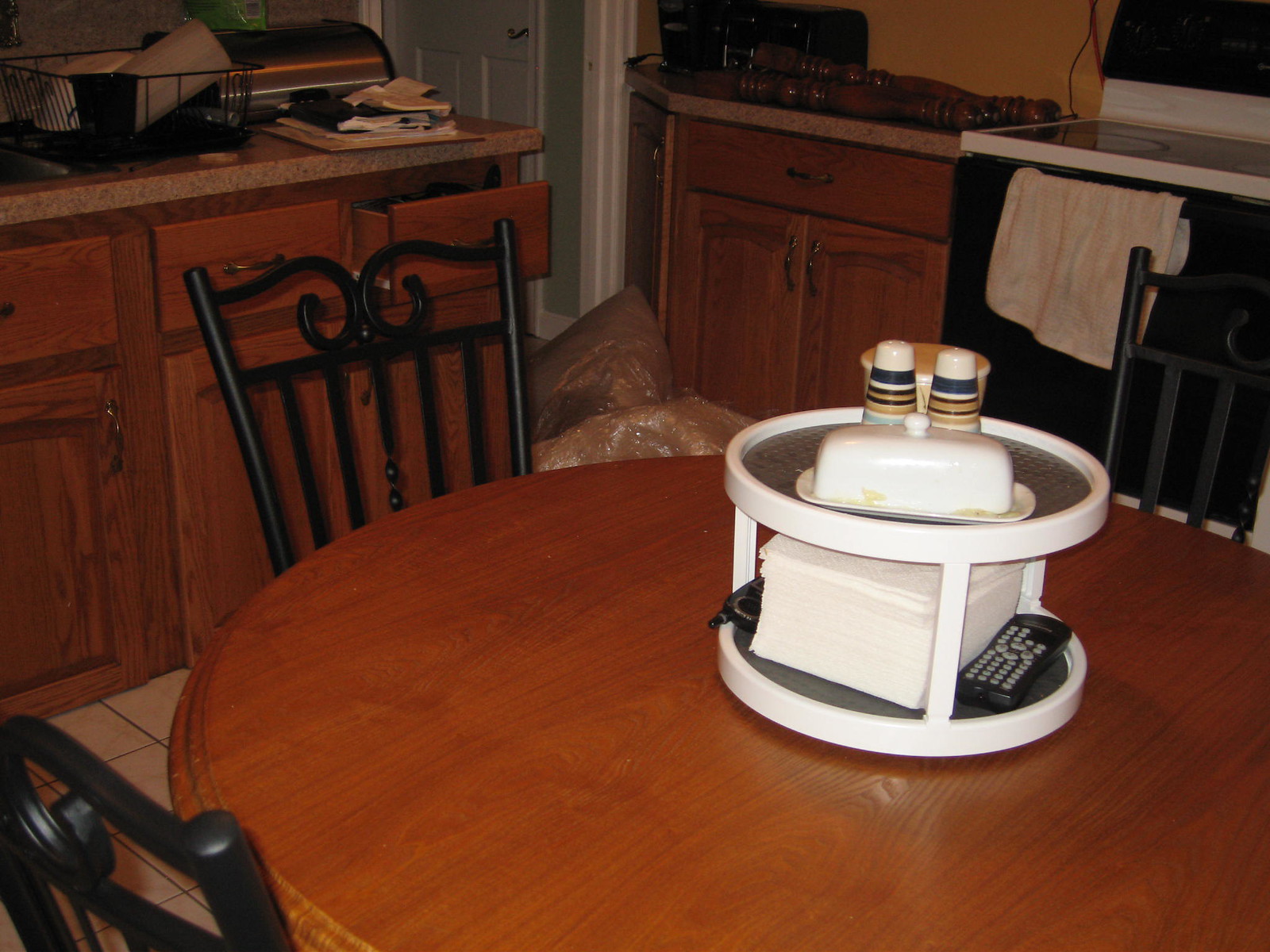The image depicts a cozy kitchen setting within a home. In the foreground, there is a circular brown wooden table accompanied by black metal chairs that sport a swirly back design. A white Lazy Susan sits atop the table, featuring a lower tier that holds napkins and is flanked by two remote controls. The upper tier of the Lazy Susan houses a white butter dish alongside salt and pepper shakers, which are adorned with black, white, and yellow stripes. Slightly obscured behind the shakers is an unidentified cup.

In the background, to the upper left, stands a black and white stove adjacent to brown wooden cabinetry. An open doorway with a green border is visible nearby. To the left of the doorway, another set of brown wooden cabinets is topped with a marble-like beige countertop. On the countertop sits a black wire dish rack with dishes inside, a stack of books or similar items, and a partial glimpse of a silver sink. The square tiles on the floor match the beige marbly color of the countertop, contributing to the overall harmonious aesthetic of the kitchen.